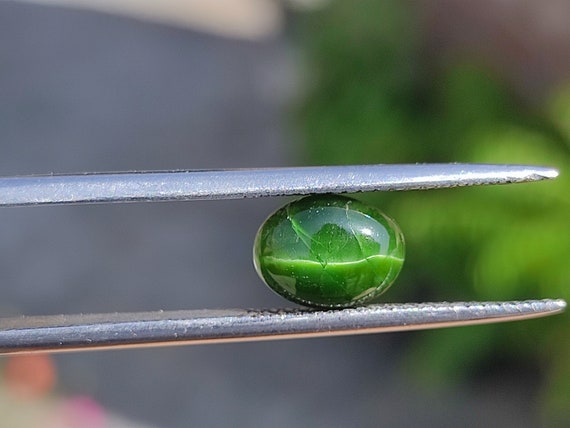The image is a close-up color photograph of a small, shiny, oval-shaped green gemstone being held by a pair of silver tweezers. The gemstone, which resembles jade or serpentine, is a glossy emerald green with a thin, wavy white line running through its center, along with a couple of other lighter cracks. Inside the stone, there is a square-shaped reflection with jagged edges and a light blue streak on the surface. The silver tweezers, designed for gripping tiny objects, feature notches on the ends for better grip and taper down towards the tips. The background is out of focus and grainy, featuring green vegetation, likely a bush, against what seems to be a rust-colored building, and some gray asphalt on the left side. In the upper left corner, a light brown, indistinct object is visible, adding to the blurred backdrop.